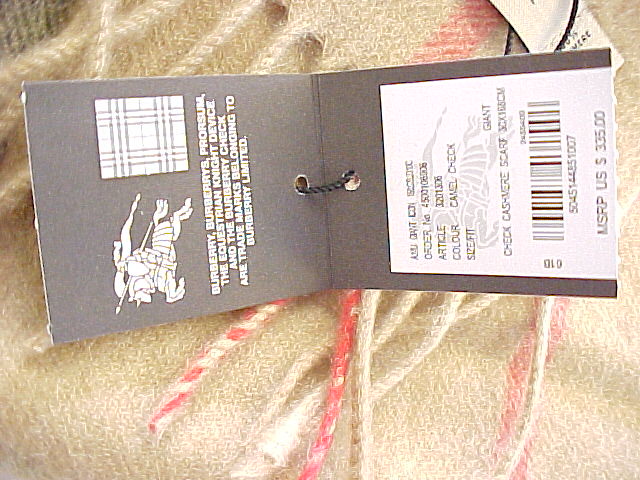A close-up photograph showcases the price tag of a luxurious Burberry cashmere scarf. The tag itself is a muted gray, secured to the scarf by a sleek black string. The text on the tag clearly indicates that it is a "Check Cashmere Scarf," with a manufacturer's suggested retail price of $335. In the background, the actual scarf is partially visible, revealing its exquisite design: a soft tan base adorned with elegant pink stripes. The fringed ends of the scarf feature an intricate blend of white and pink threads, adding to its sophisticated aesthetic. The meticulous details captured in this image suggest that it may be intended to highlight the product for potential buyers.